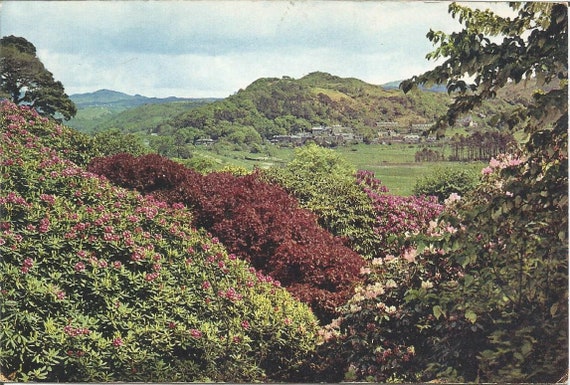This picturesque landscape photograph captures the serene and lush countryside, with expansive foliage showcasing a rich palette of red, green, pink, white, and purple hues spread across what appears to be the Welsh or possibly Italian countryside. The foreground is adorned with an array of colorful flowers—muted purple, pale pink, and dark red. Thick red and purple bushes blend into the scenery, leading the eye toward the vibrant greenery and scattered trees that characterize the rolling hills. In the distance, a quaint village or cluster of homes and villas nestles up against the looming mountains. The sky above is mostly cloudy, casting a diffused light typical of the midday in autumn. This beautiful scene stretches out for miles, emblematic of a serene, untouched valley teeming with a diverse range of plant life and very little human activity. The photograph appears to be an artistic capture, possibly a photo of a photograph or painting, lending a timeless and nostalgic essence to the imagery.